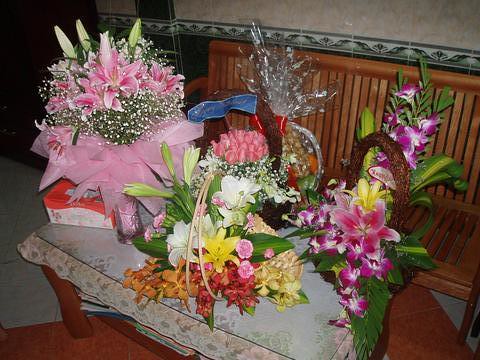This photograph showcases an elaborate display of floral arrangements set atop a wooden coffee table adorned with a white decorative cloth. The table, which also features a lower shelf holding several magazines, is positioned in front of a wooden bench, creating a warm and inviting home setting.

Prominently displayed in the front is a large light brown basket with handles, filled with a multi-colored assortment of flowers including vibrant yellow, red, orange, pink, and white blooms. To the left of this arrangement is a striking pink-ribboned container showcasing a mix of pink and white flowers, accented by small white blossoms. Next to it, an arrangement of purple orchids brings a touch of elegance with its long leaves and delicate petals.

In the middle of the table is a bouquet of various colored lilies, accompanied by three large pink and white floral bulbs that add a focal point to the composition. Behind this central arrangement is a tighter collection of approximately eighteen roses, exuding classic beauty. Toward the back is another large basket tied with a decorative bow, filled with more vibrant flowers and greenery.

On the right side of the table, a second large brown basket holds an exuberant mix of pink and white flowers, with lush green leaves spilling out, adding to the lush, garden-like feel of the display. Together, these arrangements create a mesmerizing, altar-like effect, transforming the table into a vibrant celebration of floral artistry.